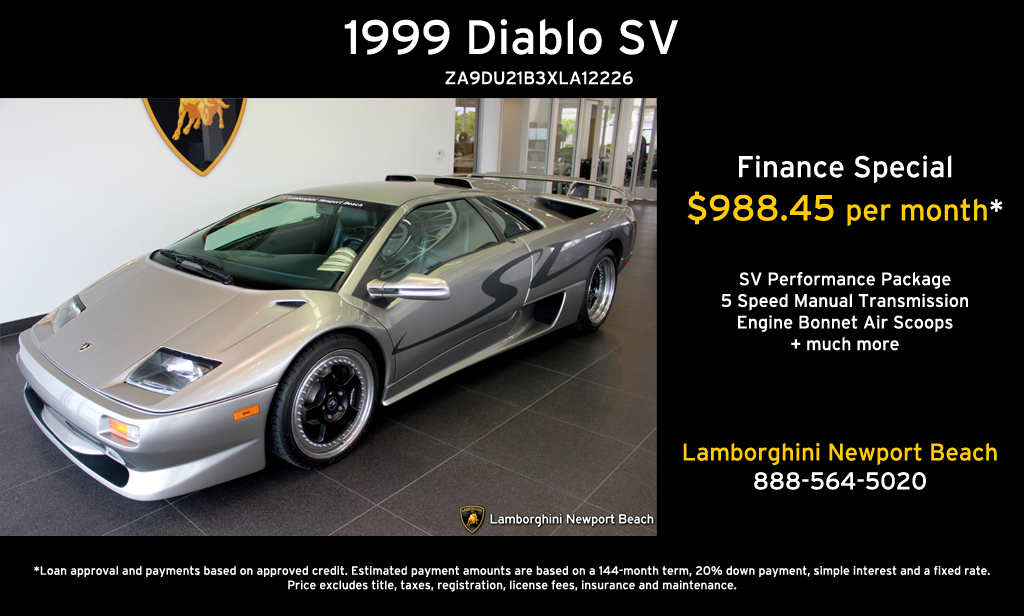The advertisement features a sleek, gray Lamborghini on a black background, prominently displaying the model and VIN: "1999 Diablo SV ZA9DU21B3XLA12226" in white font at the top. The backdrop is an authentic auto showroom with the Lamborghini Newport Beach logo and symbols adorning the walls. The car itself is positioned with its front facing the lower left-hand corner and the rear towards the upper right, set against a tiled floor with large gray squares. Details of the finance offer are specified in yellow text, highlighting a special rate of $988.45 per month, featuring an SV performance package, 5-speed manual transmission, engine bonnet, air scoops, and more. The dealership's contact information, "Lamborghini Newport Beach 888-564-5020," is provided, along with a footnote explaining that the loan and monthly payments are subject to credit approval, based on a 144-month term with a 20% down payment, simple interest, and a fixed rate. The price excludes title, taxes, registration, license fees, insurance, and maintenance.